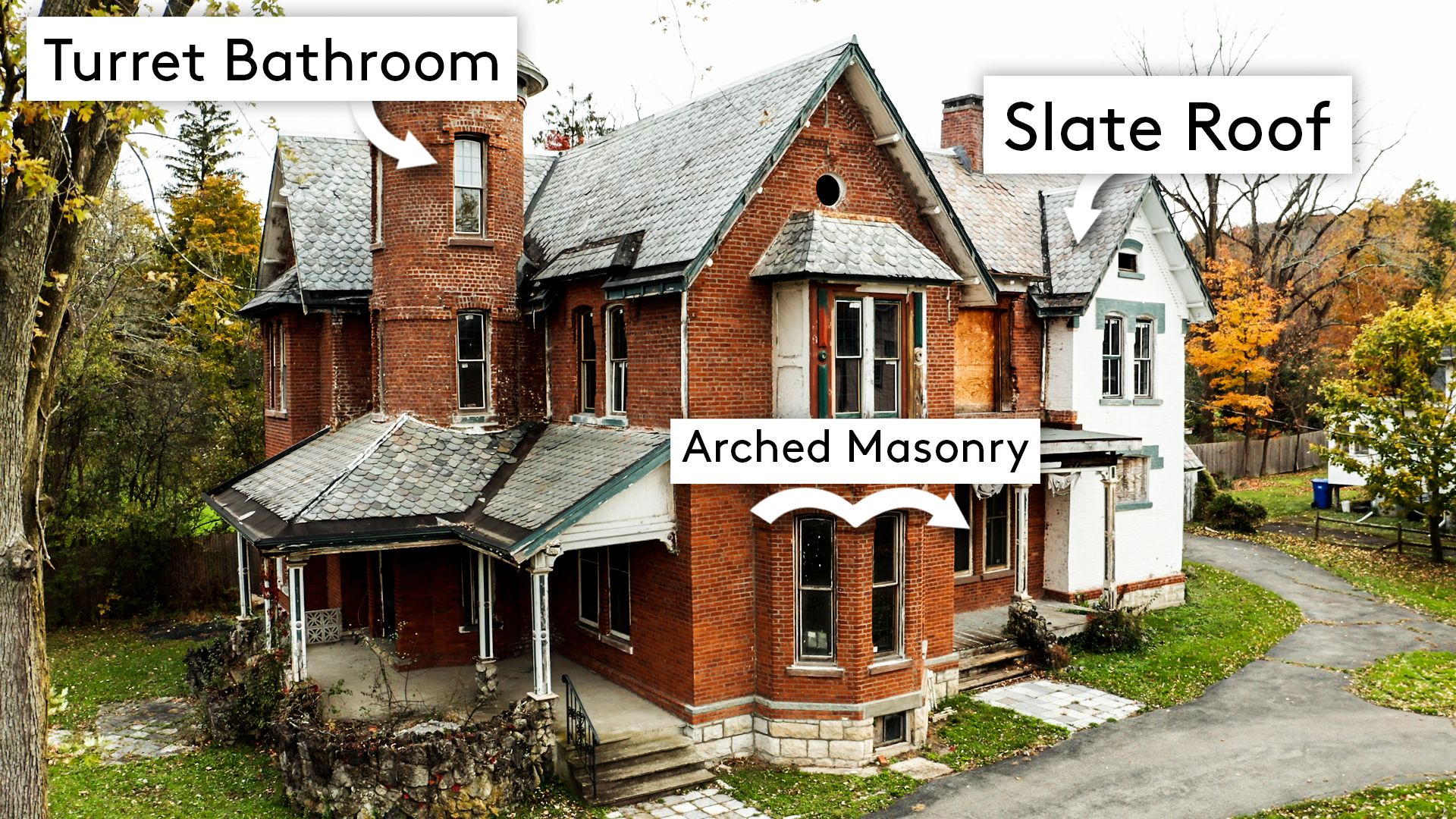The image depicts an older, large, two-story brick house with an attic, and a side addition on its right. The house features a prominent front porch and large windows. A turret with a window is located on the top floor, labeled "Turret Bathroom" with an arrow pointing to it. Another label, "Arched Masonry," arches over parts of the central structure, showcasing its architectural detail. The top right corner identifies a "Slate Roof" on the two-story white addition to the right of the main brick structure. The house is surrounded by lush greenery, including trees and plants. A walkway extends towards the right side of the house, potentially leading to additional structures or areas. The various labels and descriptive elements in the photo suggest it may be an advertisement or sale listing, emphasizing the house's unique features.